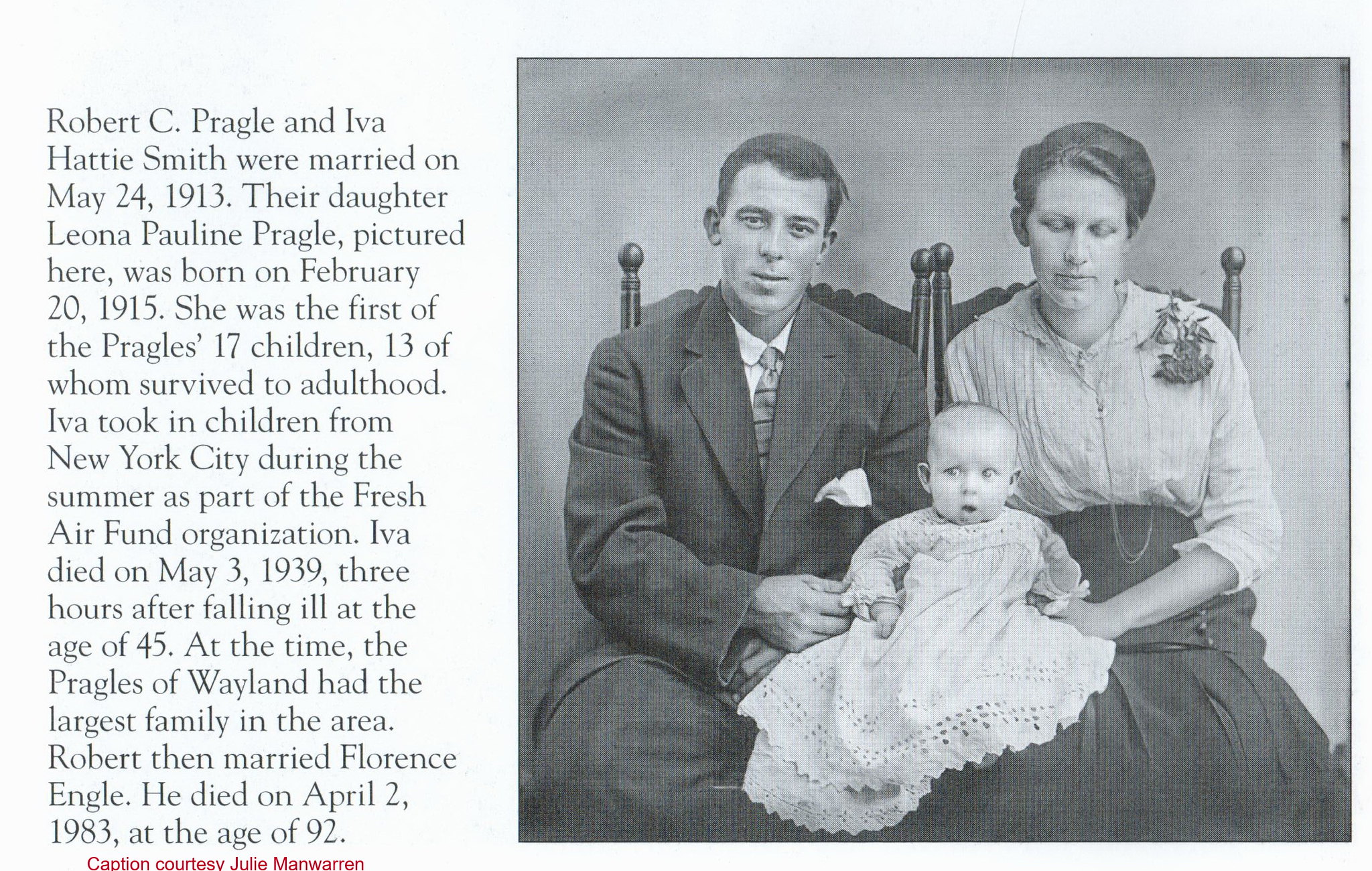This black and white photograph, likely taken in the early 1900s, features a family of three. On the left, a man with short hair wears a dark suit, appearing gray in the monochrome image. Seated beside him on the right is a woman with her hair pulled back, possibly in a bun, adorned in a white button-up shirt with elbow-length sleeves, a necklace, and a flower pinned to her left shoulder. Between them sits their baby daughter, dressed in a white lace gown, sitting upright with a slightly open mouth and sparse hair. To the left of the photograph, a text details the family's history: Robert C. Paraga and Eva Hattie Smith married on May 24, 1913. Their daughter, Liana Pauline Paragal, born on February 20, 1915, was the first of their 17 children, 13 of whom survived to adulthood. Eva, who took in children from New York City during summers via the Fresh Air Fund organization, passed away on May 3, 1939, three hours after falling ill, at the age of 45. Notably, the Paragals were known as the largest family in the Wayland area at the time. Another text indicates that Robert Henry Florets Ingle died on April 2, 1983, at the age of 92.